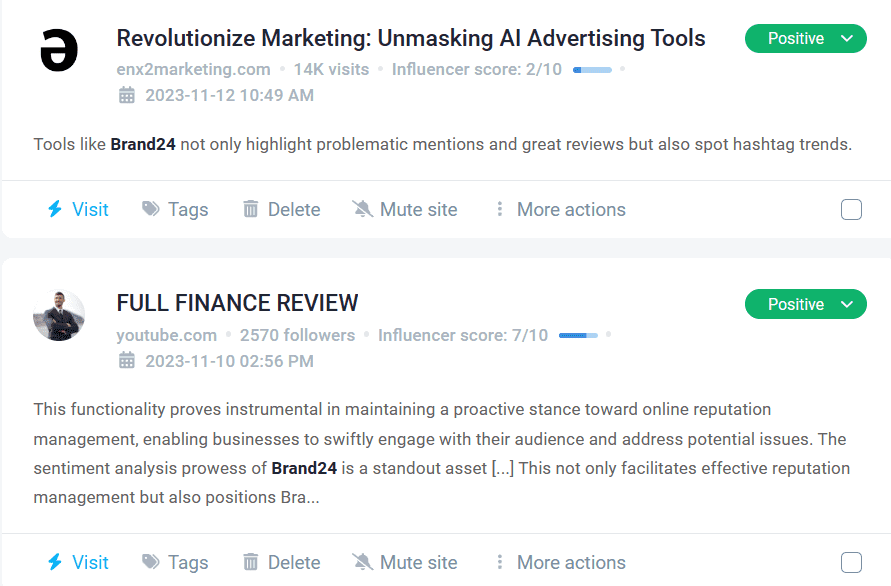Image Caption: 

The image features the title "Revolutionizing Marketing: Unmasking AI Advertising Tools" prominently displayed at the top. On the left side, there is a unique upside-down black "E." To the right, a green drop-down menu labeled "Positive" can be seen. Text within the image reads: "Tools like Brand24 not only highlight problematic mentions and great reviews, but also spot hashtag trends." Additionally, there is a blue lightning bolt icon labeled "Visit." Adjacent to this are options labeled "Tags," "Delete," "Mute," and "More Actions," followed by a white square on the far right.

Below this section, there’s a block titled "Full Finance Review," featuring a photograph of a man in a suit with his arms folded. The caption indicates "youtube.com," with a following of 2,570 people, an influencer score of 7 out of 10, and a timestamp reading "Calendar: 2023-11-10 at 2:56 PM." This positive sentiment is highlighted in green and accompanied by a drop-down arrow. The accompanying text elaborates on Brand24’s functionality, stating that it is instrumental in maintaining a proactive stance towards online reputation management. This tool enables businesses to swiftly engage with their audience and address potential issues. Notably, Brand24's sentiment analysis prowess is highlighted as a standout asset, facilitating effective reputation management. The text ends with a copyright symbol.